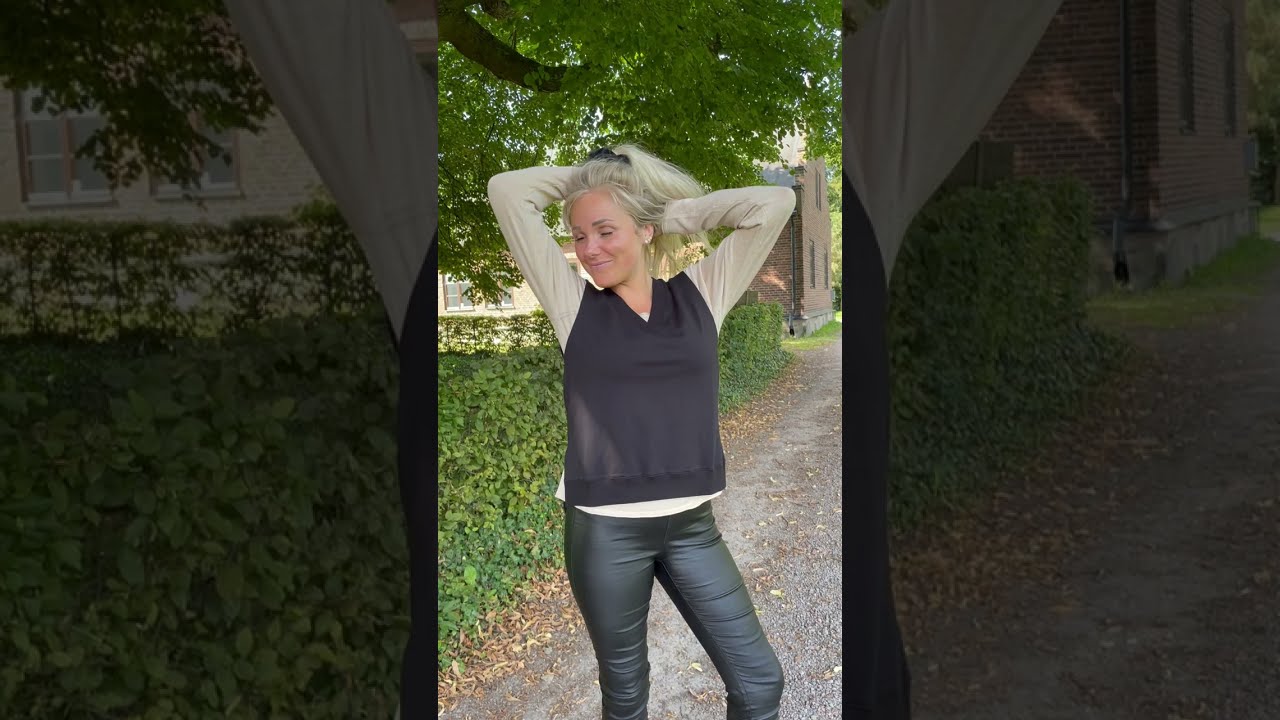The image captures a possibly middle-aged woman, likely in her 30s, posing outdoors with a relaxed demeanor. She has blonde hair with a hint of grey, adorned with a black ribbon. Her attire includes black, possibly leather, pants and a layered outfit consisting of a black vest over a long-sleeve shirt that appears to be either white or beige and gray. The woman stands on what seems to be a driveway or sidewalk, with her eyes closed and a subtle smile, as she lifts her hair with her hands positioned behind her head. The background features green plants and a large tree limb with dense green leaves above her head. Additionally, a brick building, possibly a multi-story house, is partially visible. The scene is bordered by muted elements of the main image to create a soft, grayed-out frame.